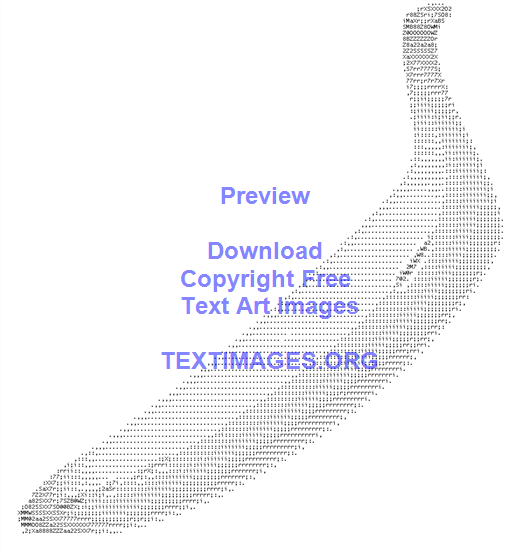The image features a perfectly shaped banana composed of numerous black dots, resembling text characters. This banana design sits prominently against a stark white background, creating a striking contrast. In the center of the image, there is blue and light purple text reading, "Preview, Download, Copyright Free, Text Art Images, textimages.org." The word "Preview" appears slightly above "Download," and there's a notable gap between "Text Art Images" and the website address. This text is neatly arranged over the middle section of the banana. The meticulous dot arrangement and the clean, minimalist background emphasize the text art's intricate design and direct viewers to textimages.org for downloading the full, watermark-free version.